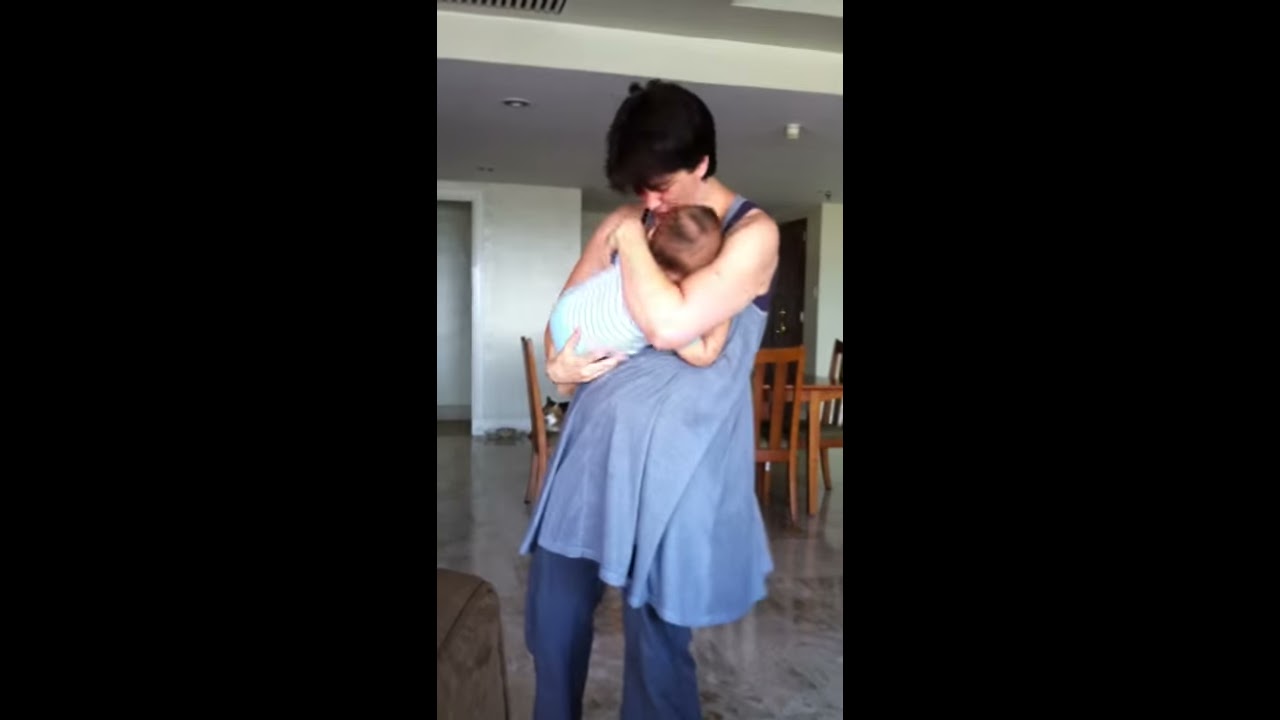In this highly detailed color photograph, we see a young woman with short black hair standing in a well-lit, modern dining room. The woman, dressed in blue jeans and a sleeveless blue tunic top, cradles an infant in her arms. She is gently bent forward from the shoulders, her gaze lovingly fixed on the baby who is nestled against her shoulder. The baby, wearing a blue and white striped onesie, looks up at her. Behind them, the dining room features polished gray marble tile flooring that reflects the surroundings, and there is a matching wooden table and chairs, each with a gray cushion. The walls and ceiling are painted white, illuminated by recessed lights, and a smoke detector is visible on the right side of the ceiling. The composition and lighting of this photograph emphasize the tender bond between the mother and child, creating a vivid and heartfelt scene.